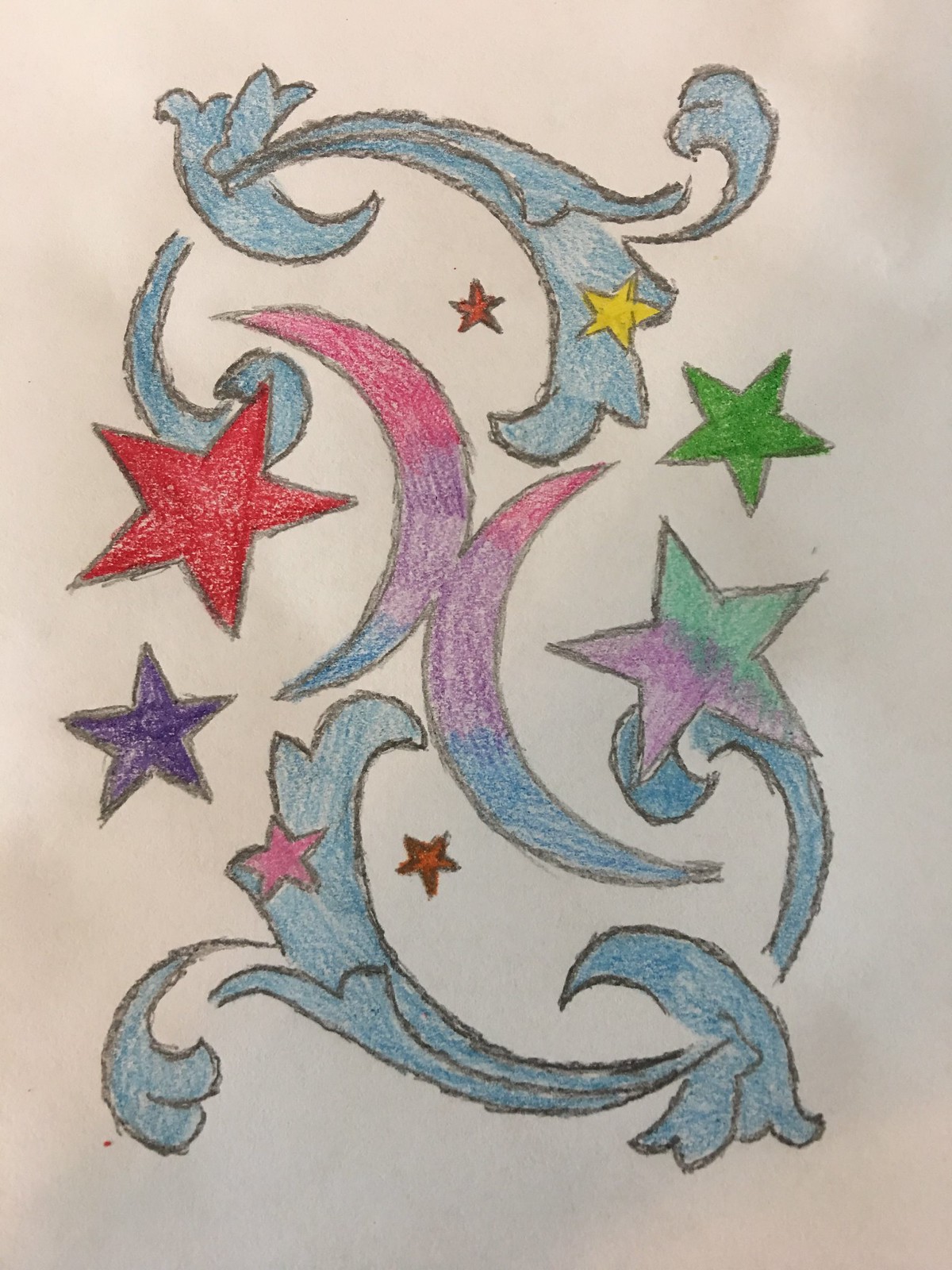This image depicts a vibrant, personalized drawing, likely a child's creation, sketched with black colored pencil outlines on cream-colored paper. Dominating the center are two conjoined half moons, oriented in opposite directions and hued in a gradient from pink at the top through purple in the middle to dark blue at the base. Surrounding the moons, a plethora of stars in various sizes and colors populate the scene: a sizeable red star, a smaller yellow star, a green star, a purple star, a star split between green and purple, and several more in shades of pink, red, and yellow. Interwoven with these celestial elements are blue swirls and wave-like or floral patterns, adding to the dynamic and whimsical composition. The colors appear lightly applied, giving the image a gentle, pastel-like softness.